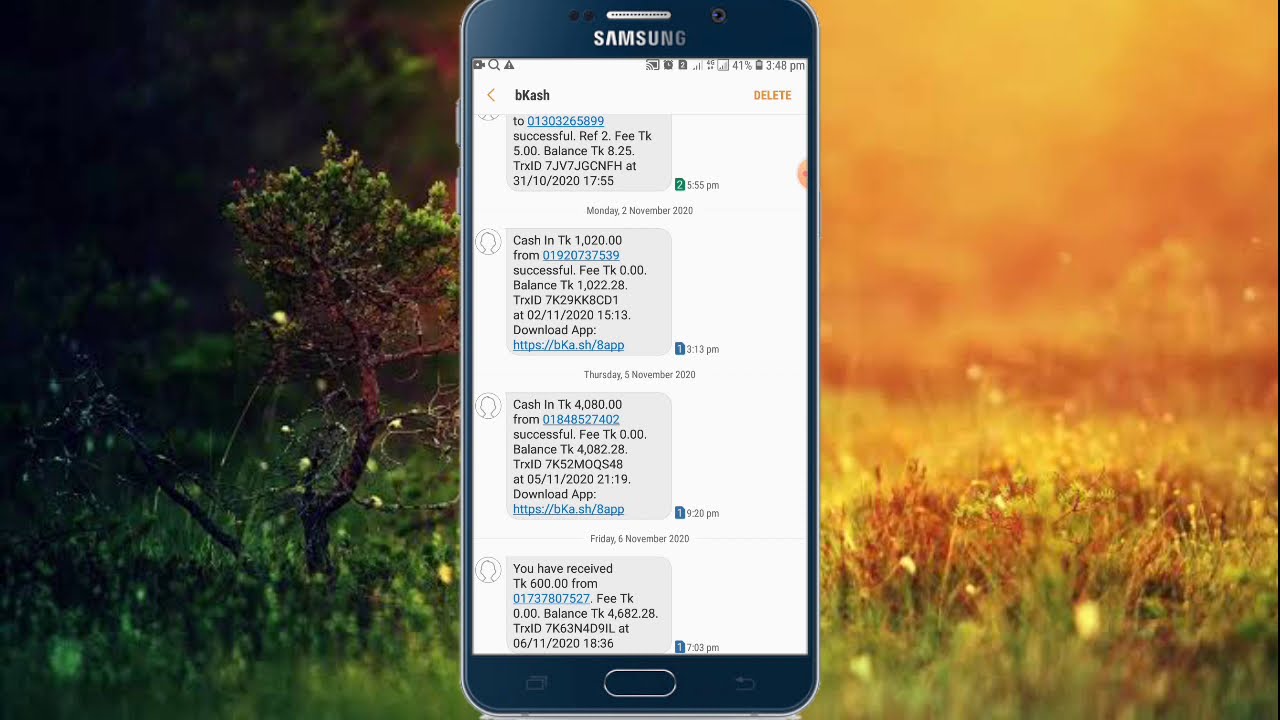The image showcases a digitally produced Samsung cell phone positioned directly in the center against a nature-inspired background featuring grass, trees, leaves, and a yellow sky. The phone screen displays a screenshot of a messaging app with four text messages detailing various transaction fees. The colorful composition includes hues of black, green, brown, white, blue, orange, yellow, and red, suggesting that this might be an advertisement for a mobile app. The natural elements and vibrant colors in the backdrop enhance the visual appeal of the scene.